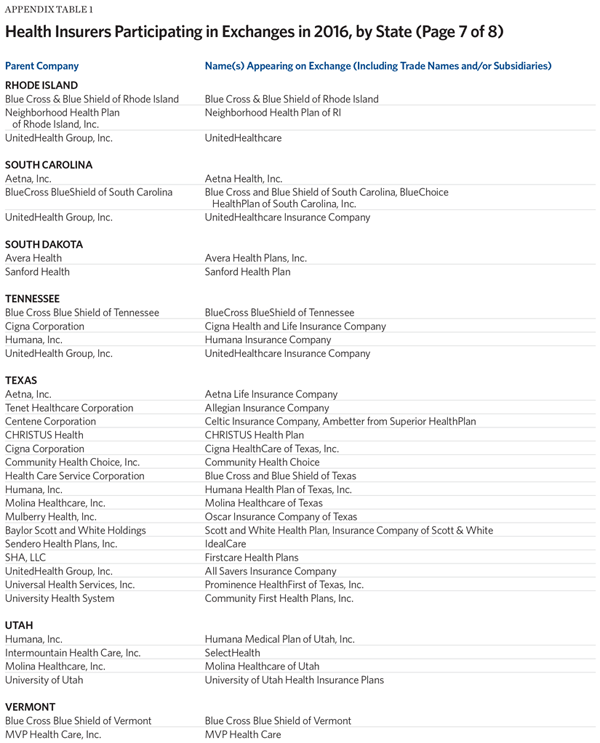This image depicts a page from a comprehensive 2016 report on health insurers participating in state exchanges. The page, identified as page 7 of 8, prominently features the title "Appendix Table 1" at the top in bold. The entire document is minimalistic, with a plain white background and devoid of any graphics.

Beneath the title, the content is organized into two primary columns. The first column, titled "Parent Company" and highlighted in blue, lists the parent companies of health insurers. The second column, labeled "Names Appearing in Exchange (including trade names and/or subsidiaries)," details the specific trade names or subsidiaries participating in the exchange.

Each state's name is presented in bold, all-caps format, marking the beginning of its respective section. For instance, Rhode Island's section lists insurers such as Blue Cross Blue Shield of Rhode Island and Neighborhood Health Plan of Rhode Island. 

Similarly, South Carolina, South Dakota, Tennessee, Texas (noteworthy for its extensive list of around 12 to 15 insurers), Utah, and Vermont follow suit. The detailed entries include insurers across various states, like Aetna Health and Everett Health Plan for Rhode Island, and Blue Cross Blue Shield of Tennessee for Tennessee.

This structured table efficiently organizes and presents the information about health insurers across different states, allowing for a clear understanding of their participation in the 2016 state exchanges.